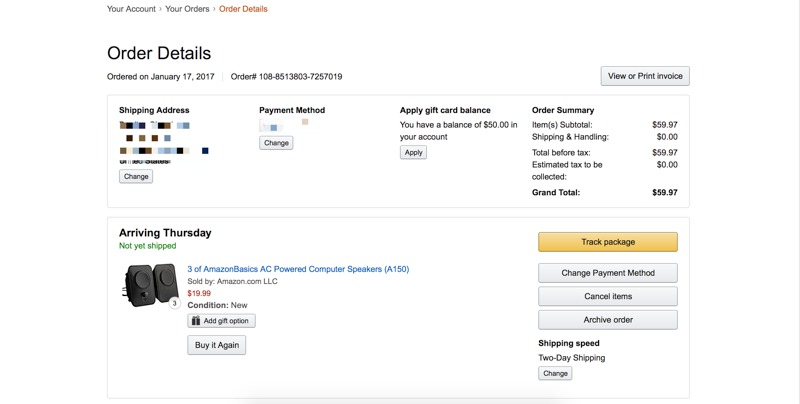The image displays an Amazon-like order details page. In the upper left corner, there is a breadcrumb navigation in smaller gray font, reading "Your Account > Your Orders > Order Details," with the "Order Details" text highlighted in orange. This indicates the current page and its navigation path.

Below the navigation trail, there are two spaces followed by the page title, "Order Details," left-aligned. Directly beneath this, in smaller font, it states, "Ordered on January 17, 2017," along with the order number. Further down, you can find sections for "Shipping Address," "Payment Method," and an option to "Apply Gift Balance."

At the bottom of these sections, the grand total for the order is prominently displayed as $59.97. Additionally, the delivery status indicates that the item is "Arriving Thursday." The ordered product is identified as AC-powered computer speakers.